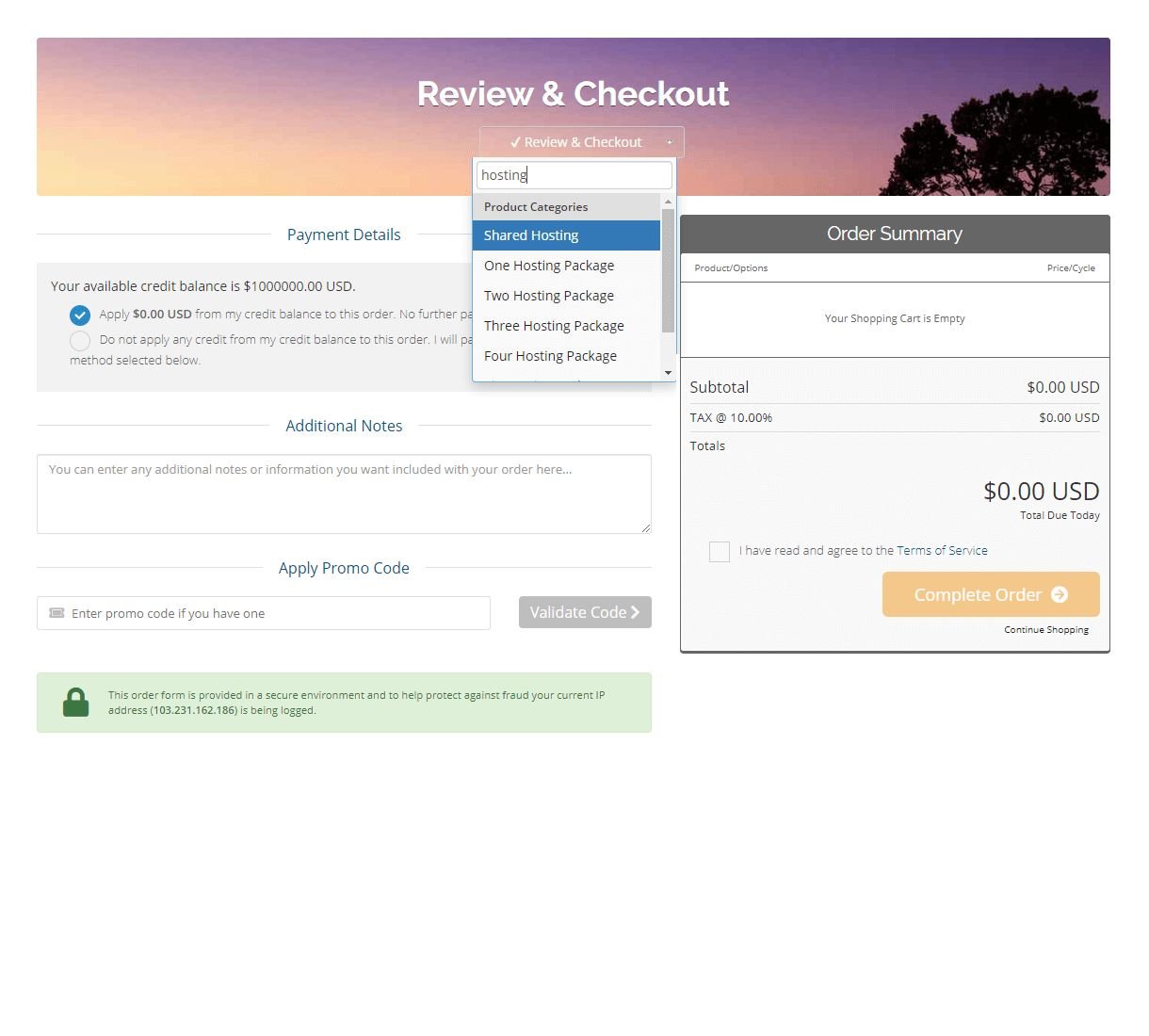Here's a refined and detailed caption for the image described:

---

The image is a screenshot of a webpage where a user needs to review and finalize a document. The page features a large horizontal banner at the top, vividly illustrated with a silhouette of a grand tree against the backdrop of a stunning sunset in hues of purple, yellow, pink, and orange. Prominently displayed in large white letters is the text "Review and Check Out." Below this banner section, the same text appears again alongside a check mark, accompanied by a drop-down menu.

The drop-down menu presents various product categories, specifically: "Shared Hosting," "One Hosting Package," "Two Hosting Package," "Three Hosting Package," and "Four Hosting Package." The "Shared Hosting" option is highlighted in blue, indicating the user's current selection. Additionally, the user has typed "hosting" in the search box.

On the left side of the page, there is a section titled "Your Available Credit Balance," showing a balance of $10,000,000, though without commas. A checkbox below this section states "Apply $0 from my credit balance to this order" and is marked with a blue checkmark. Underneath, another option reads "Do not apply any credit balance," but this box remains unchecked.

Further down, there is an "Additional Notes" field where users can type additional information or instructions. A "Promo Code" section invites users to enter a code in a text box and validate it by clicking a gray button next to it.

On the right, the "Order Summary" reveals that the shopping cart is currently empty, displaying a subtotal of $0, tax of $0, and a total of $0. The page concludes with a prominently placed yellow button labeled "Complete Order."

---

This caption comprehensively details the content and layout of the webpage as described.